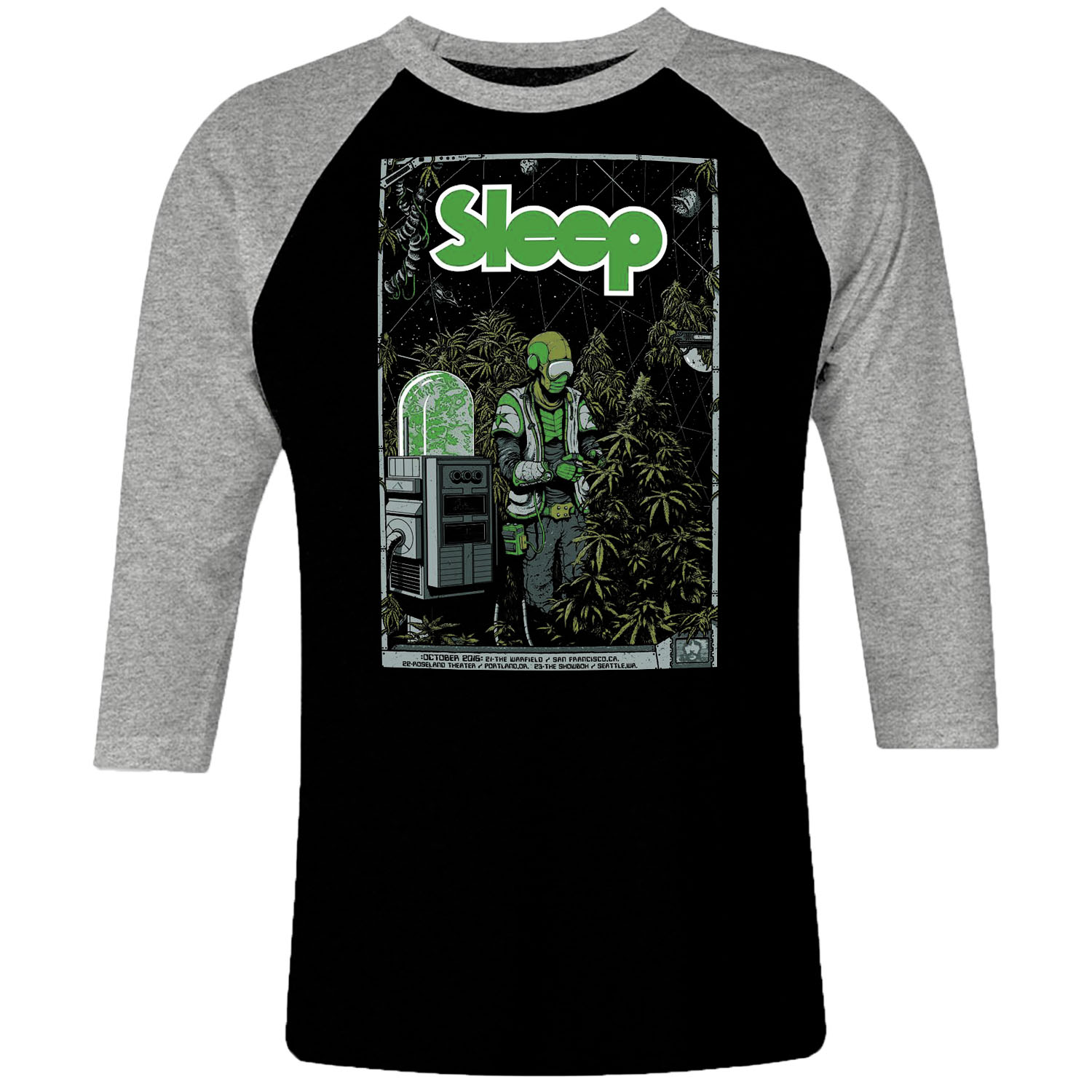This image features a three-quarter length sleeve baseball-style t-shirt displayed against a white backdrop. The shirt's body is black, while the sleeves and neckline are a light gray. The front of the shirt showcases a tall rectangular design outlined in white. Prominent within this design is the word "sleep" in large green text. Below this text, there is an image of a person dressed in green suit armor, resembling a gardener or worker, wearing a vest, helmet, and goggles. They appear to be interacting with plants and bushes beside a machine with a dome top containing a green substance. The scene is lush with foliage and the detailed design creates a vivid narrative. At the bottom of the design, there is fine print that includes the date "October 2016" among other hard-to-read text.